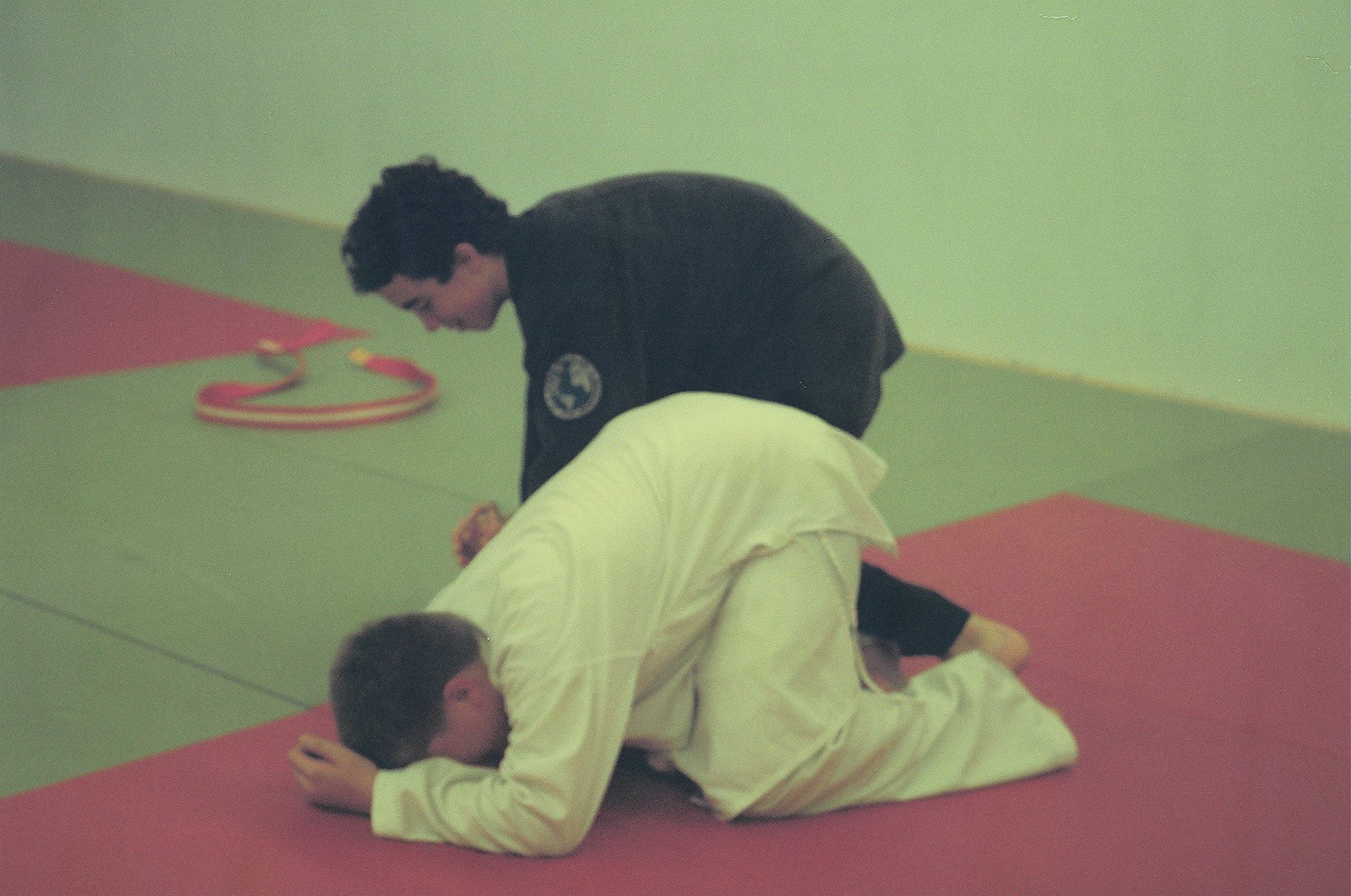In this detailed photograph, two young men, likely teenagers, are engaged in a martial arts practice or competition inside a room with green walls. The floor is covered with gray and red mats, and the specific area where they are situated features a prominent reddish-colored mat. The young man in the foreground is dressed in a white gi and is positioned with his elbows and knees on the mat while his head is bent down, making his face mostly obscured by the mat. He appears to be in a distressed position, as if struggling in the bout. Behind him, his opponent wears a black gi with an emblem that resembles the earth in off-white on his arm. The opponent is also bent over but remains partially upright, smiling slightly. Both boys have short hair and are barefoot. Noticeably, a belt, possibly red with a white stripe, lies on the mat, though it is somewhat blurry in the image. The scene is set against a backdrop of additional mats and what appears to be a white wall, highlighting the intensity and focus of the ongoing practice or competition.